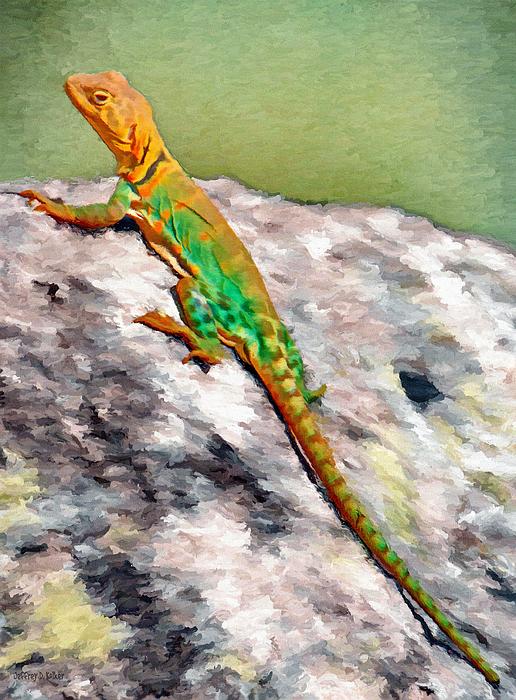The image depicts a detailed painting of a vibrant forest scene. Dominating the foreground is a large, multifaceted stone that spans roughly four-fifths of the canvas, presenting a subtle spectrum of grays, light whites, and hints of light purple. Atop this textured rock rests an intricately colored iguana. The iguana stretches diagonally from the lower right to the upper left corner, its head positioned upwards towards the left. The creature’s body showcases a vivid palette: the head is a striking burnt orange, transitioning into a mix of green and orange along its back and legs, and further adorned with yellow and green, striped with orangish-brown, trailing down its lengthy tail. The backdrop features patches of lush, lime and darker green foliage, suggesting the forest surroundings. This combination of natural elements and vibrant wildlife conjures an immersive and lively outdoor setting.